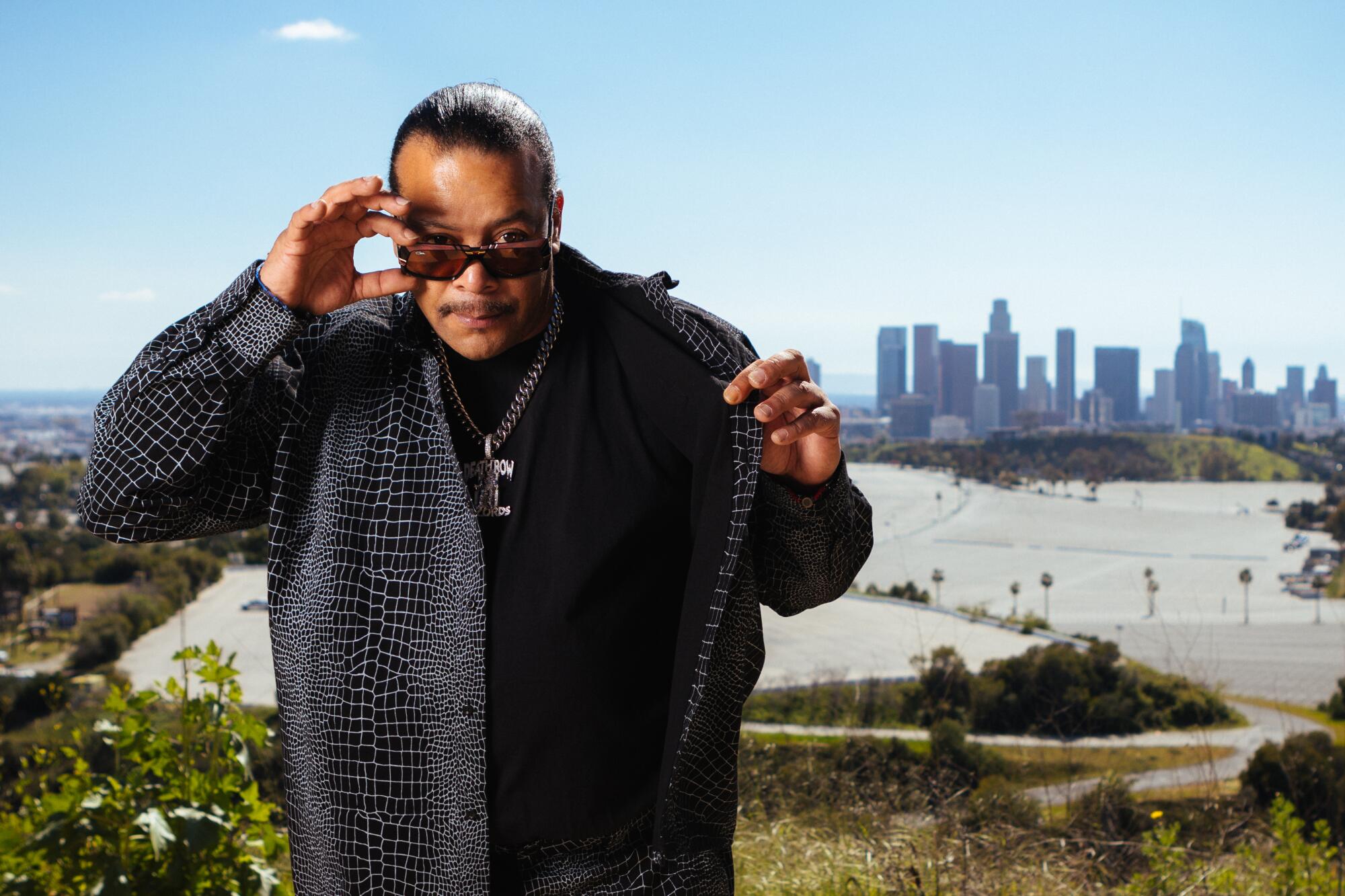The photograph features a man of mixed-race heritage, possibly Hispanic or Hispanic-Asian, with a dark complexion and slicked-back brown hair, accentuated by a receding hairline. He sports a brown mustache and is peering over his brown sunglasses with a subtle smile. The man is dressed in a distinctive outfit that includes a gray-black, snake-patterned jacket, a black top, and a striking silver chain necklace with "Death Row Records" partially inscribed on it, hinting at a hip-hop connection. His right hand opens the jacket to reveal the chain, while his left hand adjusts the sunglasses on his nose.

The image is set outdoors during the daytime, likely for a promotional shoot, with the man standing at the top of a hill. The background showcases a sprawling cityscape of Los Angeles dotted with skyscrapers, palm trees, a white landscape, and smaller houses to the left. The setting also includes hints of a parking lot area and various roads leading up to the elevated spot where the man stands, surrounded by plants and grass.